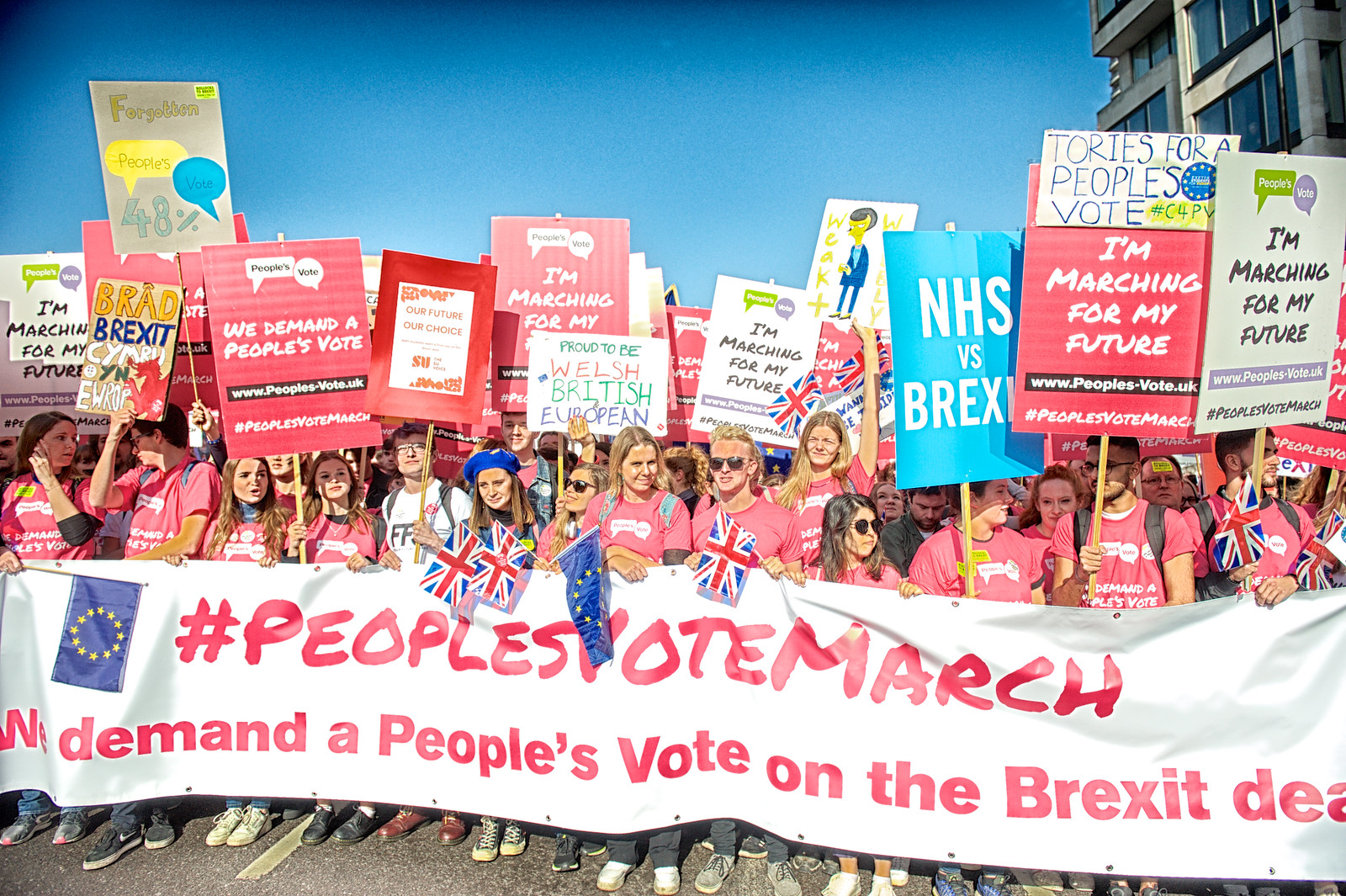In this detailed photograph of a protest, a large and diverse crowd of young adults, consisting of both men and women, are gathered in the center of an outdoor setting. The protestors are standing on asphalt pavement, indicative of a regular road, with multiple buildings visible in the background on the right side of the image. The crowd is prominently visible, vividly dressed mostly in pink shirts with speech bubbles containing the text "People's Vote" and additional messages that read "We Demand a People's Vote."

At the forefront of the protest, the first line of individuals is holding a substantial white banner with striking red text that reads "People's Vote March." Below this, it states "Demand a People's Vote on the Brexit Deal." The crowd is holding a variety of signs, both printed and handmade, featuring slogans such as "We Demand a People's Vote," "NHS vs Brexit," "Tories for a People's Vote," "Our Future, Our Choice," "Bad Brexit, Simri YN EWROP," "Forgotten, People's Vote, 48%." Some protestors are also waving British and European Union flags, demonstrating the group's diverse yet unified call for a referendum on the Brexit deal. The protest appears to be taking place in the middle of the day and is part of a larger march advocating for change.